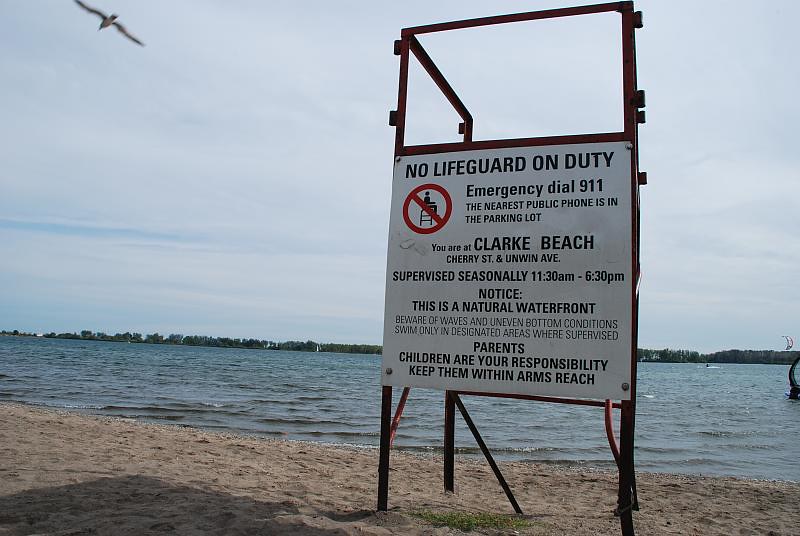The image depicts a horizontally aligned rectangular picture of a beach scene. Dominating the sandy foreground is a large, white warning sign mounted on black metal poles. The sign features several messages in black print, starting with "NO LIFEGUARD ON DUTY" at the top, followed by an icon of a lifeguard chair with a red circle and slash through it, indicating absence of lifeguard services. To its right, it states, "EMERGENCY DIAL 911," and notes that "The nearest public phone is in the parking lot." Further down, it identifies the location as "CLARK BEACH," with an address at Cherry Street and Owen Avenue. The sign also mentions supervision hours, "seasonally from 11:30 a.m. to 6:30 p.m.," and provides a safety notice about it being a natural waterfront along with a warning for parents to keep children within arm's reach.

The softly choppy water behind the sign has gentle waves more akin to a lake than an ocean, with a tree-lined horizon in the distance. In the upper left-hand corner of the image, a large bird, blurred from motion, is flying with its wings spread. The sand is light tan, and the background extends to a clear blue sky, emphasizing the tranquility of the scene.